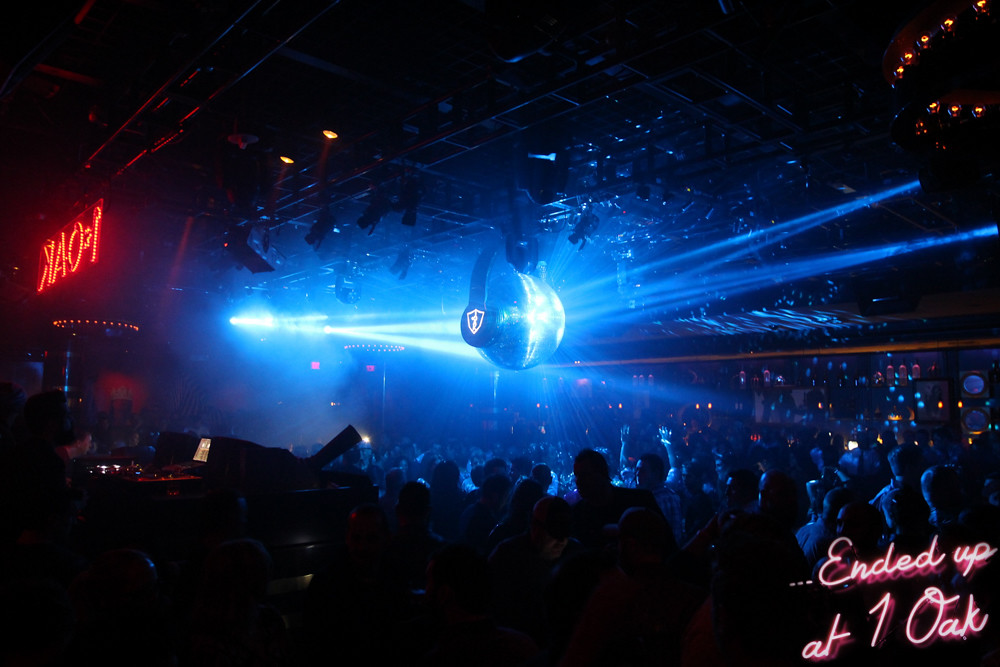The image captures the vibrant scene inside a dimly lit nightclub. Dominating the center is a large mirrored disco ball, shimmering in various shades of blue from lights cast upon it, with prominent white streaks emanating towards the ball from the left. Beneath this centerpiece, a crowd of people on the dance floor has their hands raised in celebration, immersed in the electrifying atmosphere. In the upper left corner, a red and yellow neon sign reads "One Oak," albeit reversed, appearing as "K-A-O-1" from this angle. A semicircular string of yellow lights adorns the upper right section, adding to the festive display. To the left, a DJ booth is visible with a DJ orchestrating the music and light show. In the lower right corner, in pink lettering, the phrase "...ended up at One Oak" caps off the scene, reflecting the attendees' exhilarating experience.